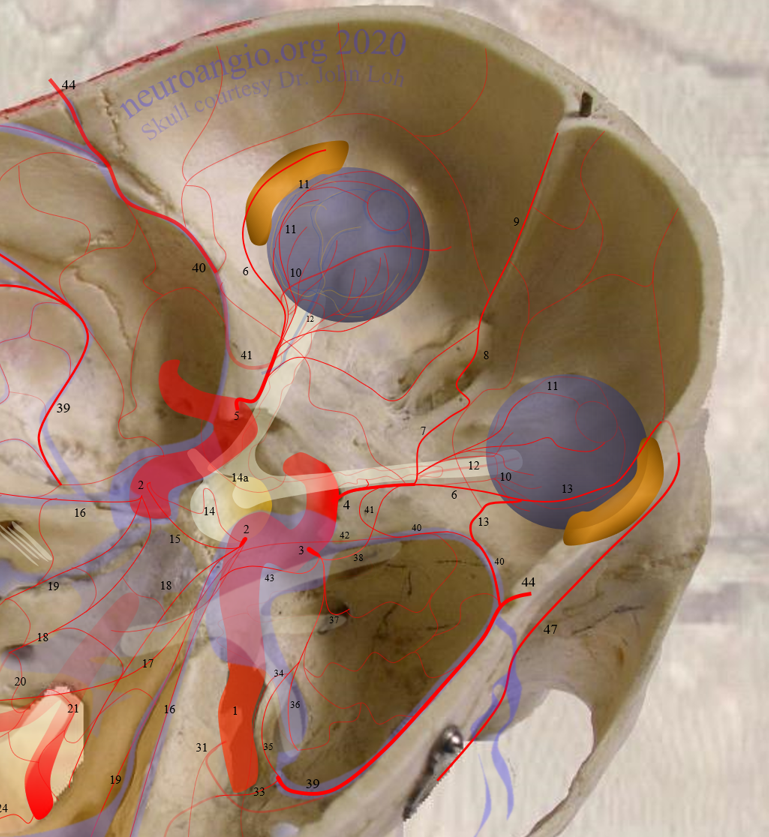The image depicts a halved skull, courtesy of Dr. John Loh, for neuroangio.org 2020. It is displayed on a whitish, water-stained gray background, and measures 8 inches wide by 9 inches tall. The text "neuroangio.org 2020" is seen at the top in dark purple lettering alongside "Skull Courtesy of Dr. John Loh."

The skull features metal connectors to allow it to be reassembled. It is digitally augmented with a superimposed diagram highlighting the locations of veins and nerves, particularly around the optic region. Eyeballs and visual dynamics are indicated with numbered placements in black, including numbers such as 2, 10, 11, 14a, 16, 17, 20, and 41. However, the numbers and color codes lack a correlating key for detailed understanding.

Throughout the image, various colored elements are present: football-shaped yellow and gold structures, blue circles with smaller orange entities, and red squiggly lines resembling fine blood vessels and worms. These anatomical and artistic details lend a vivid, somewhat abstract quality to the depiction, underscoring its scientific and educational purpose.